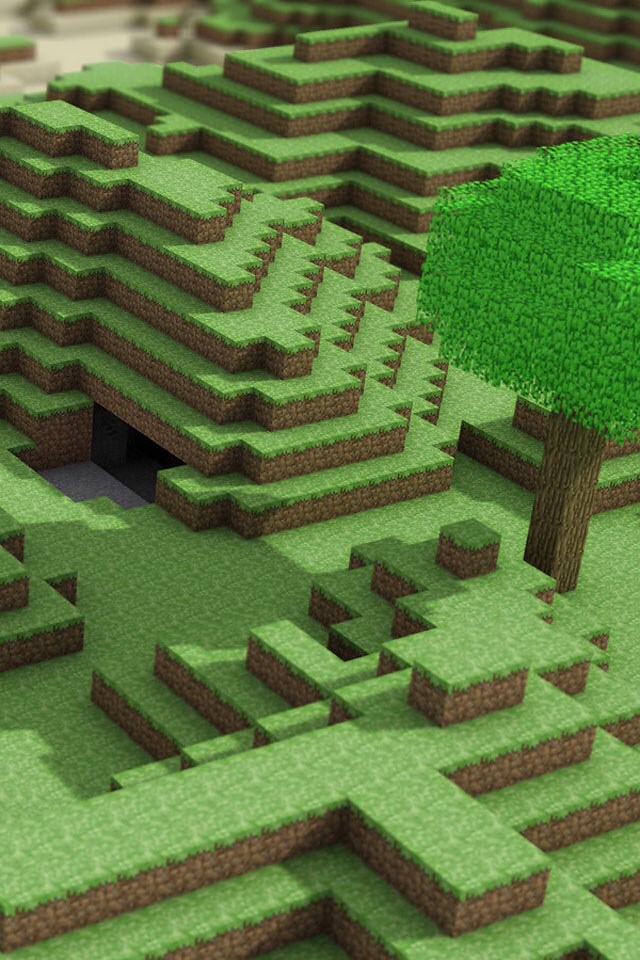This vibrant and pixelated image appears to be a screenshot from the popular video game Minecraft, depicting a richly detailed, blocky landscape. Dominating the scene is a grassy plain with hills or a mountain-like formation, entirely composed of pixel-like grass blocks with green tops and brown dirt bottoms. To the left, nestled among the grass, is a dark gray stone patch adjacent to a black-looking wall, adding a textured contrast. The right side of the image features a striking tree with a distinctly brown block trunk and bright green blocky leaves, affirming the pixelated, block-built aesthetic that is characteristic of the game. In the background, towards the left, there's a glimpse of a sandy terrain, further accentuating the diverse yet cohesive blocky environment. Each element of the image, from the landscape to the tree, exemplifies the iconic blocky, pixelated style of the game.